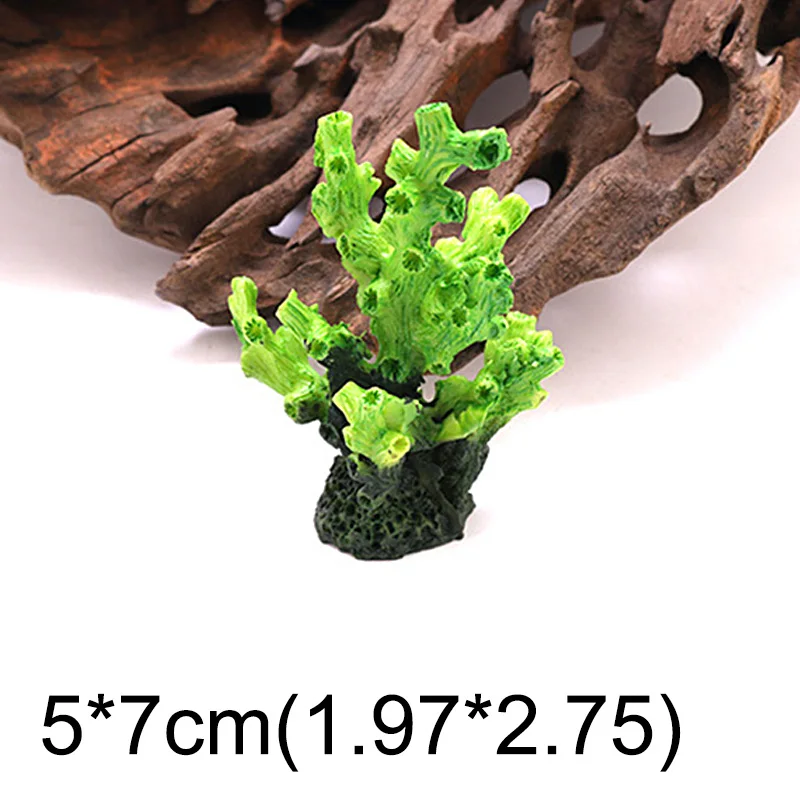This image features a detailed close-up of a small piece of vivid green coral, with a dark green to brown base. The top part of the coral is composed of tendril-like, branching structures that extend upwards, resembling tree branches. These structures are light green, transitioning to a darker green, and include sub-branches that are only a few millimeters in length, adding a complex texture to the coral. The background is a stark white, which makes the subject stand out prominently. Positioned behind the coral is a large piece of driftwood, characterized by its dark, reddish-brown color and hollow, dome-like shape with multiple holes. This wood structure takes up a significant portion of the background, offering a contrasting backdrop to the coral's bright green hue. At the bottom of the image, a large black text reads the dimensions "5 x 7cm (1.97 x 2.75 inches)," clearly indicating the size of the coral piece. The combination of these elements creates a vivid, detailed depiction of the coral against a simple white background.